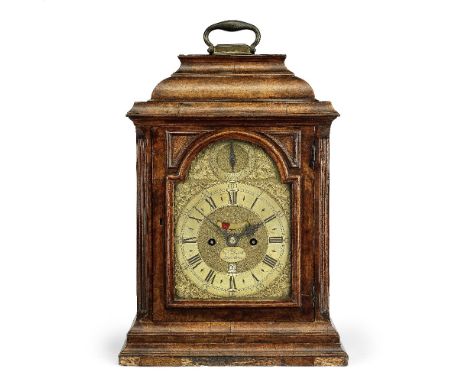This image features an antique-style wooden clock, reminiscent of a Grandfather clock but designed on a smaller scale, suitable for a tabletop. The clock is crafted from dark, high-quality wood that exhibits a washed and slightly discolored finish, highlighting its aged aesthetic. It features a prominent handle or latch at the top, likely for carrying or securing the clock. The clock face is adorned with Roman numerals and has a yellowish-gold hue. Above the clock face, there is an intricate design, possibly resembling a compass, adding to its elaborate detail. The background of the image is white, which accentuates the fine craftsmanship and ornate features of the clock.